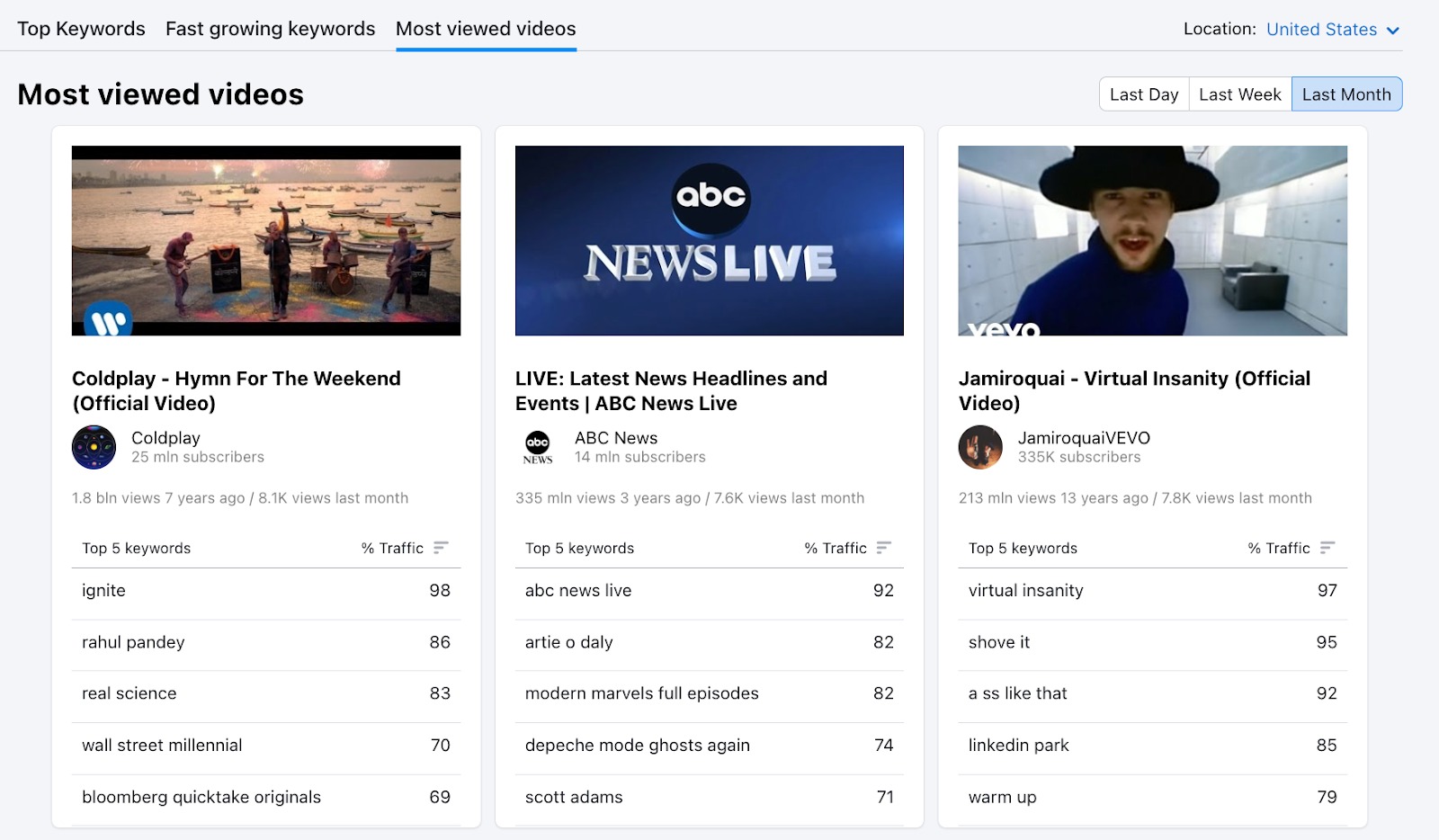The image depicts a website's search engine interface. At the very top, there are three tabs labeled "Top Keywords," "Fast-Growing Keywords," and "Most Viewed Videos." On the left side of the interface is the word "Location," next to which "United States" is displayed in blue with a downward arrow beside it. This suggests that the location is selectable.

Beneath the interface's header, a blue line under the "Most Viewed Videos" tab indicates it is the active selection. To the right, the words "Most Viewed Videos" are prominently displayed. To the left of this text, there are three filter tabs labeled "Last Day," "Last Week," and "Last Month." The "Last Month" tab is highlighted in blue, denoting it as the current filter in use.

Below these filters, the interface showcases three different content squares. The first square highlights the video "Hymn for the Weekend" by Coldplay, indicating it as one of the most viewed videos. Adjacent to this, another section lists the top five keywords associated with these popular videos. The content includes mentions of "ABC News Live," and another video titled "Jamiroquai - Virtual Insanity (Official Video)" is also featured with its corresponding top five keywords displayed below.